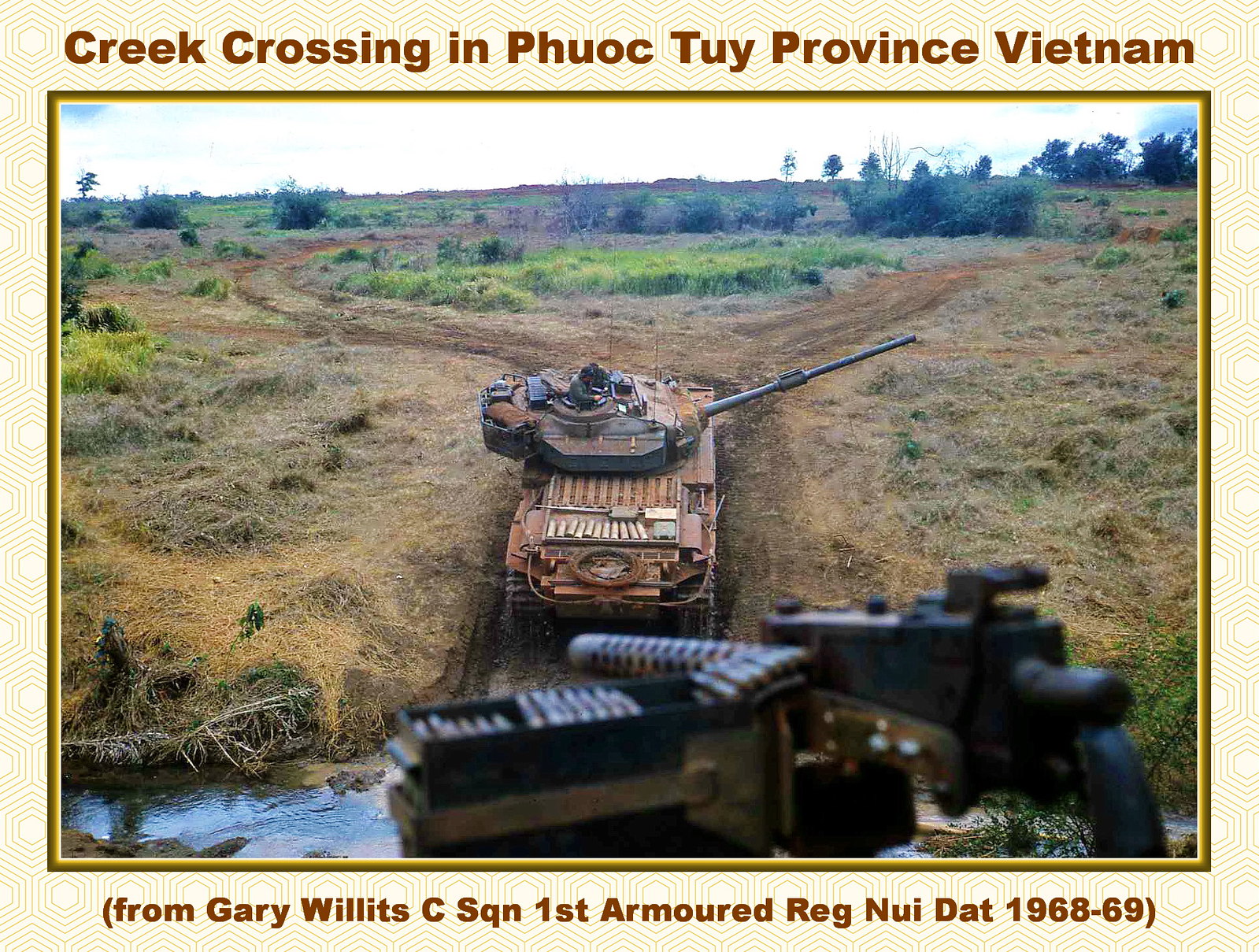The image is a historical postcard titled "Creek Crossing in Phuoc Thuy Province, Vietnam." It features a central armored tank, distinguished by its rust-brown metal hue, in the act of emerging from a stream. The surrounding environment is a mixture of green and dead grass, giving the appearance of a rugged battleground. The scene includes two diverging dirt roads ahead of the tank, leading off to the right and left respectively. The backdrop is dotted with trees, enhancing the rustic and dirty landscape. In the foreground, slightly out of focus, is a machine gun, suggesting that the photograph was taken from behind it. Notably, the bottom border of the postcard credits the image to Gary Willits, C-Squadron, 1st Armored Regiment, with the date specified as 1968-69, adding a personal and historical context to the powerful scene.